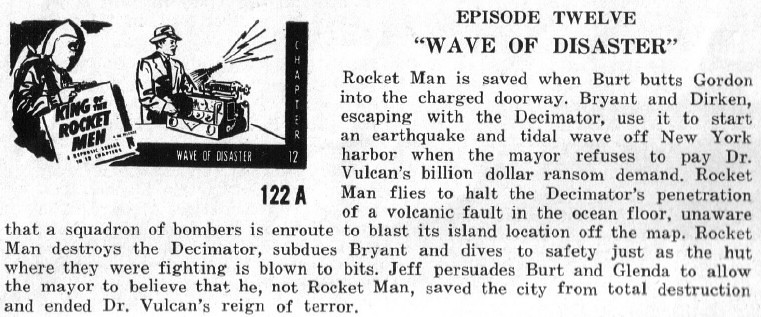The image seems to be a text-heavy page, likely from a book or magazine, featuring a black-and-white illustration on the top left that depicts a man in a hat and suit interacting with a radio device emitting radio waves. Next to him, there is another figure in a mask holding a sign that reads "King of the Rocket Men." The illustration captions include "Wave of Disaster" and "Chapter 12," with an identifier "122A" beneath it.

The text on the image, titled "Episode 12: Wave of Disaster," describes an action-packed sequence in which Rocket Man is initially saved when Bert butts Gordon into the charged doorway, allowing Bryant and Durkin to escape with the Decimator. They plan to use it to trigger an earthquake and tidal wave in New York Harbor after the mayor refuses to meet Dr. Vulcan's billion-dollar ransom demand. Rocket Man intervenes to stop the Decimator from penetrating a volcanic fault on the ocean floor. Meanwhile, a squadron of bombers is dispatched to destroy the island where the Decimator is located. Rocket Man ultimately destroys the Decimator, subdues Bryant, and escapes just as the hut they're in explodes. Lastly, Jeff convinces Bert and Glenda to let the mayor believe that he, not Rocket Man, was the hero who saved the city and ended Dr. Vulcan's reign of terror.